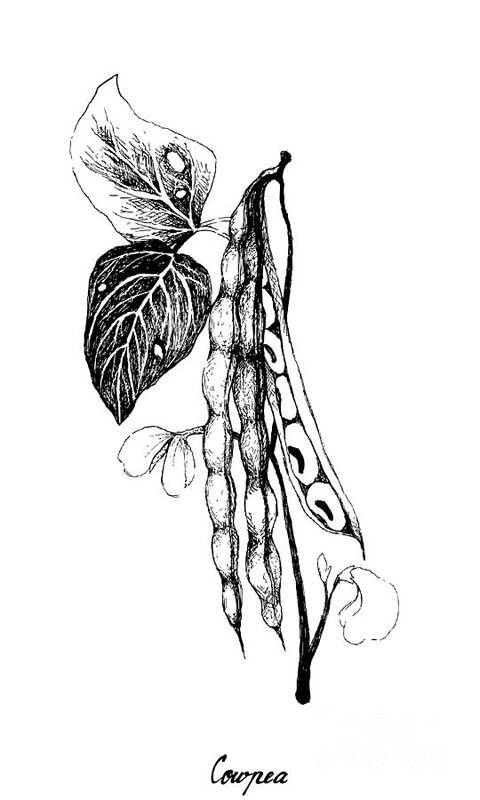This black-and-white drawing depicts a cowpea plant against a white background. The central stem, which is textured in black, supports three pea pods. Two of the pods remain intact, while the third is sliced open, revealing the peas inside. The peas resemble black-eyed peas, with a light exterior and a darker spot in the center. The plant also features two large leaves at the top—one black with pronounced white veins and the other white with subtle black accents and detailing. Both leaves display intricate vein patterns and small holes, possibly from bug bites. Additionally, the illustration includes two delicate blossoms: one situated towards the bottom right and another in the middle. The drawing is signed at the bottom with the word 'cowpea' in cursive, with a capital 'C' followed by lowercase letters.